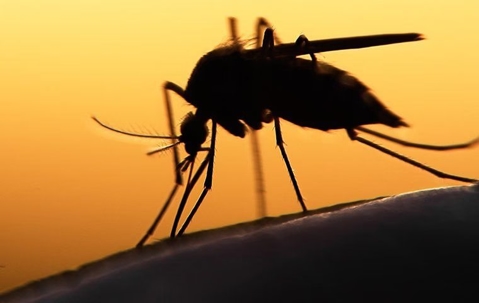This detailed close-up image features a mosquito-like insect, with a striking backdrop of an out-of-focus, gradient sunset transitioning from yellow at the top to orange. The mosquito, which could also be mistaken for a bee due to its relatively thick body and hunched posture, is perched on a solid black surface that appears to be a part of a person or animal. The insect's small head is directed downwards, revealing two large antennae and a straw-like proboscis, possibly in the act of feeding. Its elongated, straight wings extend from its back, and it has six legs visible in the image. The lighting casts the mosquito in a silhouette, emphasizing its shadowy form against the vivid sunset hues behind it.